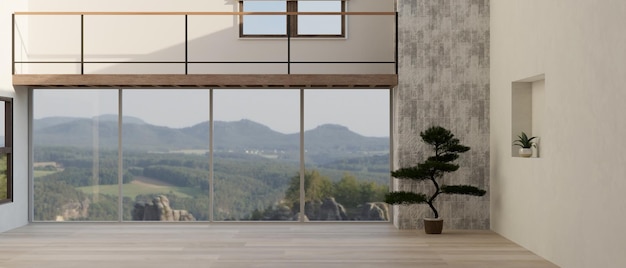The image depicts the interior of a spacious and modern home with a blend of Victorian and Scandinavian design elements. Dominating the left and center areas of the room are four large paneled windows that offer a breathtaking view of rolling hills, mountains, and scattered trees in the wide-open landscape beyond. On the right side, a white wall features a square cutout housing a potted succulent, adjacent to which is a grey textured accent panel displaying a large potted tree. Moving towards the center of the room stands a notably tall bonsai tree. An internal balcony with a beige railing, featuring square cutouts, runs above the windows. This upper level includes additional windows with brown paneling that match another window on the left side, which is slightly visible. The flooring in the room consists of high-end wooden planks, accentuating the modern yet cozy atmosphere of the living space.